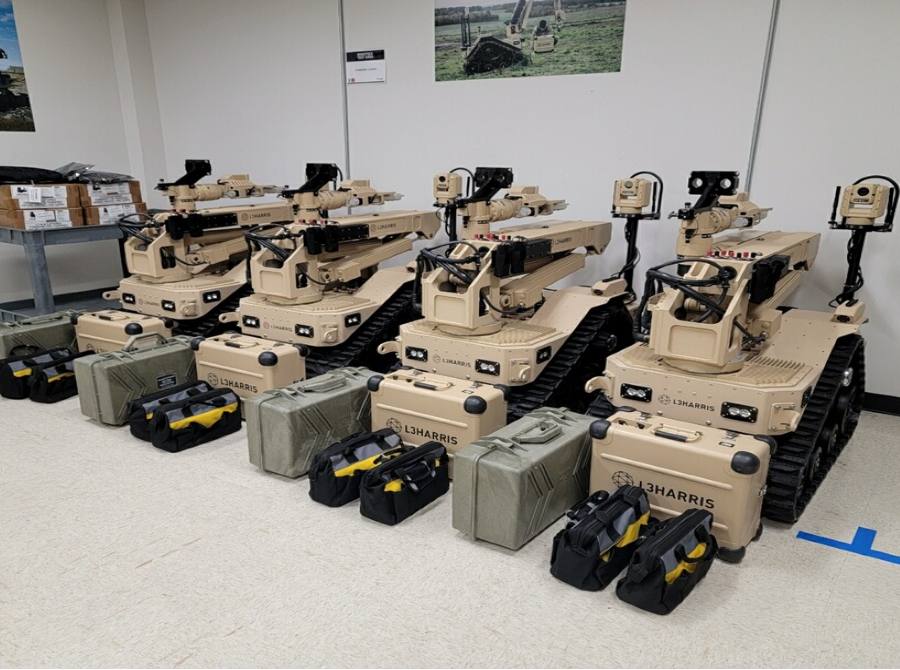The photograph captures a detailed scene of multiple small, military-style robotic vehicles lined up meticulously against a white wall within a rectangular room. The flooring consists of white tiles, emphasizing the orderly arrangement of the tan-painted, box-like robots. Each robotic vehicle is equipped with black tracks instead of traditional wheels, giving them a tank-like appearance. Mounted on the backs of these vehicles are large cranes and black poles holding cameras, with numerous wires extending from each. The robots have "I-3 Harris" labeled on the front, and are adorned with various gadgets on top.

A colorful poster on the wall behind them shows the robots in action in a green field, adding context to their purpose. In front of the vehicles lies a large, matching tan-colored crate bearing the same "I-3 Harris" marking, accompanied by two smaller gray and teal equipment cases, as well as multiple black, gray, and yellow equipment bags. This well-organized setup, framed by a white wall and tile floor, underscores the precision and purpose of these advanced, tan-colored military robotic machines.